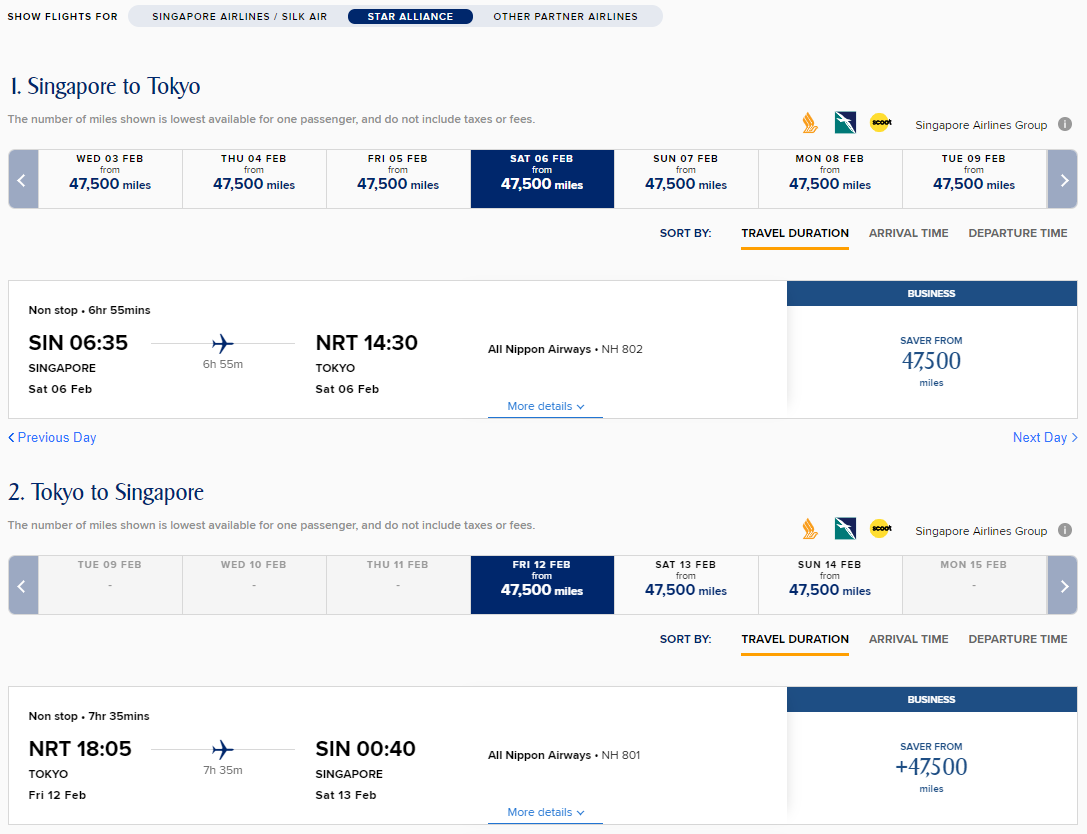The image depicts a flight schedule for a round trip from Singapore to Tokyo. The background is predominantly white with black text for clarity. At the top of the schedule, the route "Singapore to Tokyo" is displayed, followed by travel dates listed from February 3rd to February 9th in small horizontal boxes. The date "Saturday, February 6th" is prominently highlighted in dark blue with white text. Below this, flight details specify a departure from Singapore at 6:35 AM and an arrival in Tokyo at 2:30 PM. To the far right, a note indicates that business class saver seats are available starting from 47,500 miles.

The second part of the schedule outlines the return flight from Tokyo to Singapore, with dates from February 9th to February 15th shown in similar small boxes. The date "Friday, February 12th" stands out in dark blue with white text. The flight details for this date indicate a departure from Tokyo (NRT) at 6:05 PM, arriving in Singapore early the next day at 4:40 AM, on Saturday, February 13th. Again, to the right, a note indicates that business class saver seats for this leg also start from 47,500 miles.